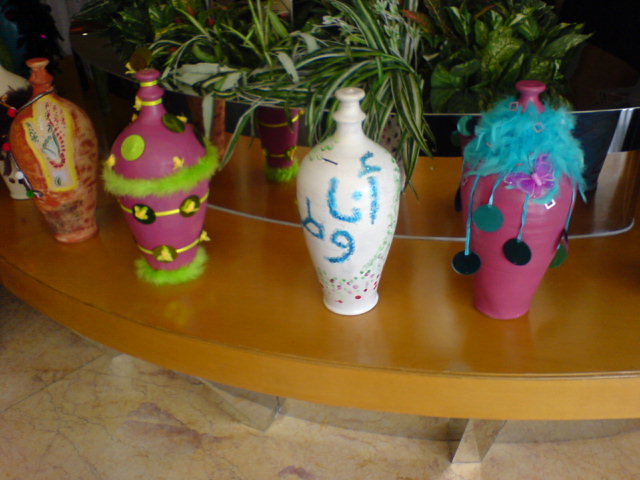The image depicts a collection of four distinct vases, each uniquely decorated, arranged on a light, caramel-colored, round wooden table with metal legs. Behind the table stands a large mirror reflecting part of the room, with a verdant plant featuring long green leaves with white streaks placed centrally in the background.

On the far left, an ornately decorated orange vase showcases a prominent right handprint outlined in yellow, with intricate red and green patterns inside, including a red snake-like design.

Next to it, a purple vase has a furry bottom and a furry ring around its mid-section, adorned with yellow stripes and black circular designs that contain detailed drawings. 

The third vase is primarily white, embellished with blue text and a pattern of pink and blue polka dots.

Furthest to the right, a purple vase stands out with blue yarn at its top, from which dangle three large dots—two black and one bluish-gray—suspended by blue strings. The marble floor beneath features a light gray base with subtle purple and yellow streaks, adding a sophisticated touch to this artistic arrangement.